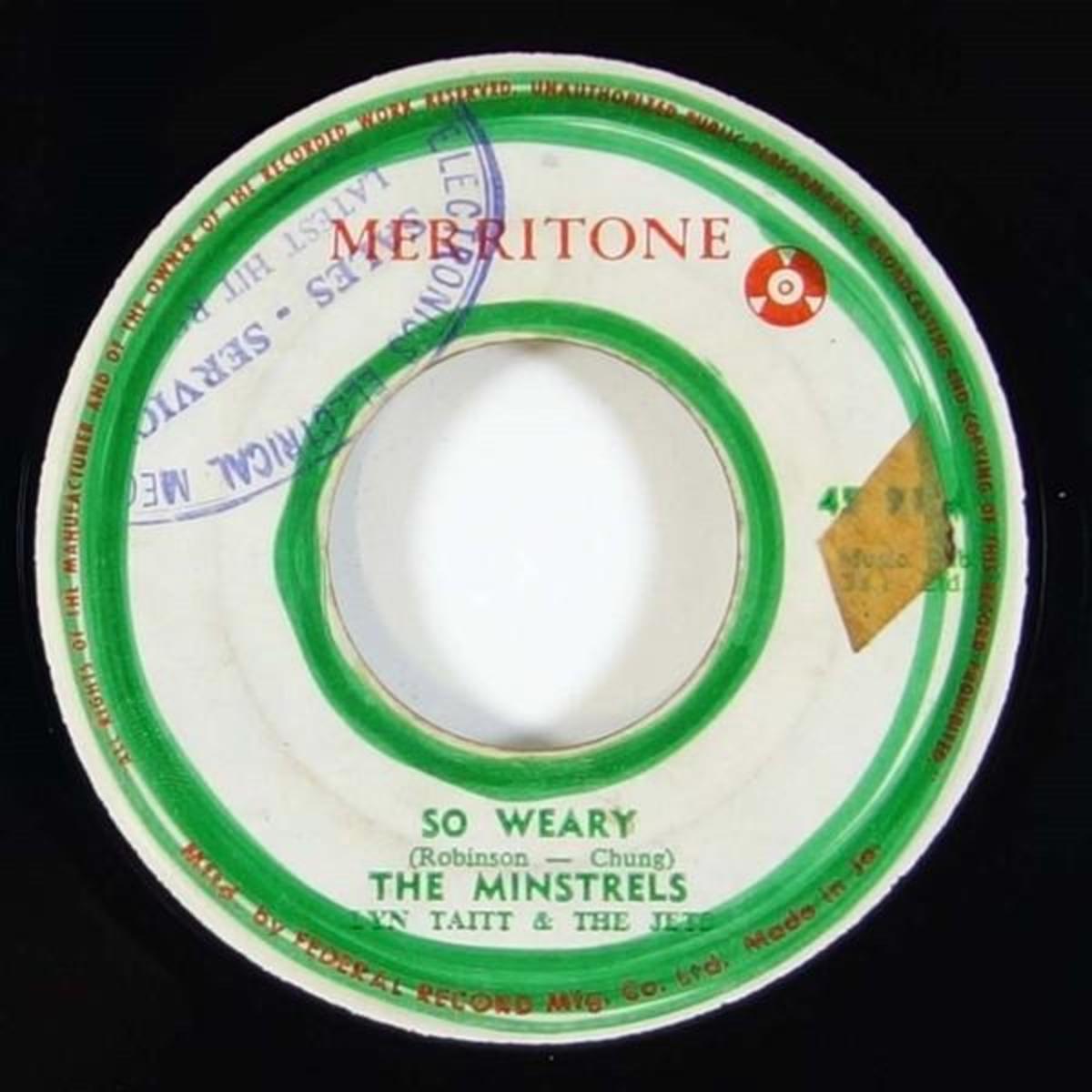The image is an up-close photograph of a worn and aged vinyl record label. The record label is predominantly white with bright green trim around the perimeter and center. At the top center, in bold red text, it reads "MERRITONE" with a small emblem resembling a record or a lifeguard float to its right. Just below, in green text, it says "SO WEARY" followed by "Robinson-Chung," "The Minstrels," and "Lynn Tate and The Jets." Surrounding the label, in red text, are various copyright notices, though some of the text appears blurred and difficult to read. There is a notable piece of dirty, aged masking tape on the right side of the label, and a blue oval hand-stamped mark that says "ELECTRONICS ELECTRICAL SALES SERVICE LATEST HIT." At the very bottom, in small red text, it states "Manufactured by Federal Record and Manufacturing Company Limited."